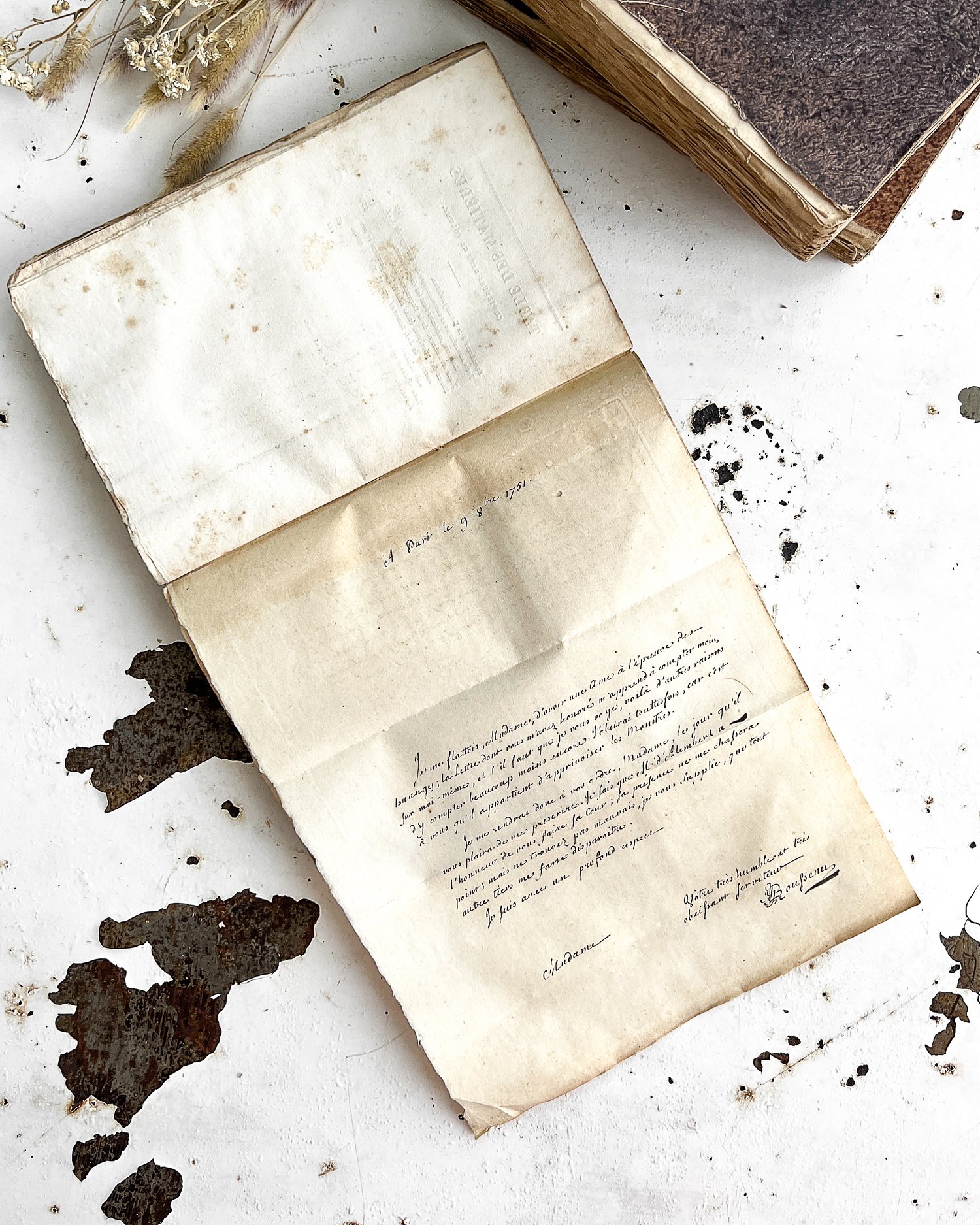The image depicts an open book resting on a weathered, white-painted wooden surface characterized by chipped paint and dark brown areas, especially at the bottom left. The book is oriented such that one side is positioned at the upper left of the frame, descending diagonally to the right. Instead of a typical book page opposite the crease, there's a letter that also slopes down to the right, seemingly attached but not confirmed. The visible page of the book is a faded yellowish color with faint black handwriting in a foreign language, resembling a journal entry or note. The open book and letter highlight their aged condition with water spots and wear reflecting their historical character. Adjacent to the main book, at the upper right corner, part of another book or journal's spine can be seen, with a dark brown cover atop a lighter brown one. Above the books, there's dried sage or grass-like flowers resting gently on the surface, enhancing the image's rustic and vintage appeal.